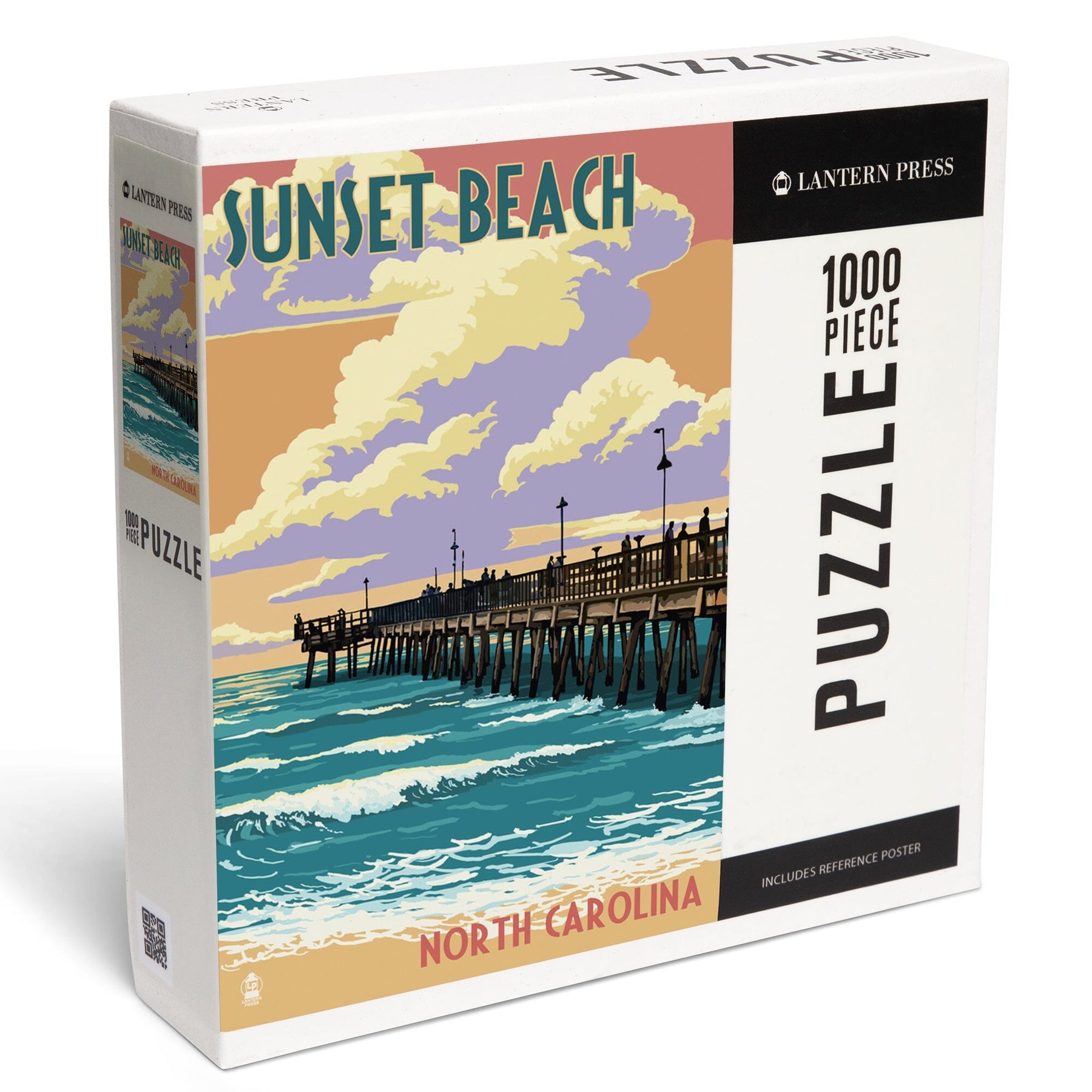The image showcases a predominantly white puzzle box containing 1,000 pieces. The box features a detailed illustration on the front, resembling a hand-drawn postcard of Sunset Beach, North Carolina. The artwork includes a boardwalk and dock extending into a teal ocean with gentle waves, set against a vivid sky painted in shades of purple, orange, pink, and cream, along with soft white clouds. At the top left corner of the front face, "Sunset Beach" is prominently displayed in large black letters, while "North Carolina" is written in reddish-pink text in the middle. The brand "Lantern Press" appears in the top right corner within a small black box, as well as in another black box at the bottom, which also appears to contain some additional text. The phrase "1,000 piece puzzle" is repeated in black text on all sides of the box. A QR code is visible on one side, emphasizing the interactive element of the product. The overall design creates an inviting visual of a picturesque beachscape at sunset, neatly packaged for puzzling enthusiasts.